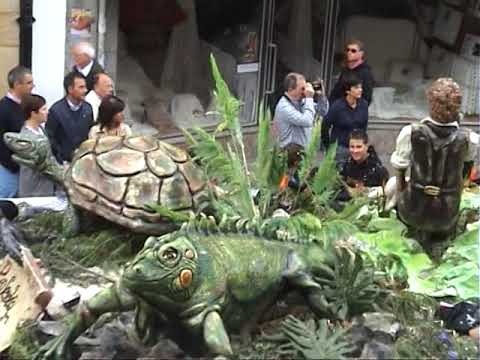The image portrays a lively parade taking place on a narrow, possibly European street lined with aged stone and plaster buildings showing signs of wear. The focus is a grand float adorned with intricate statues, the most prominent being a large, sculpted head of an elderly man with a long, white beard and flowing hair, reminiscent of Christopher Lee’s portrayal of Saruman from "The Lord of the Rings." This head has deep wrinkles and a solemn expression. Alongside this central figure, the float features statues of horses, possibly demonic figures, and other indistinct elements, such as a body in the Vitruvian Man pose. The float is draped in blue fabric around its base.

The street is bustling with activity; numerous people in white shirts walk alongside the float, helping guide it through the route. Onlookers crowd the sidewalks, watching the spectacle with interest. The parade moves through what appears to be a very old section of town with visible cracks and decrepit railings, adding to the historic charm of the scene. The atmosphere is overcast, with participants dressed in long sleeves and pants, indicating a cooler season. From the elevated angle of the camera, the image captures not only the float but also the multitude of parade participants extending into the distance, creating a vivid and detailed snapshot of this celebratory event.